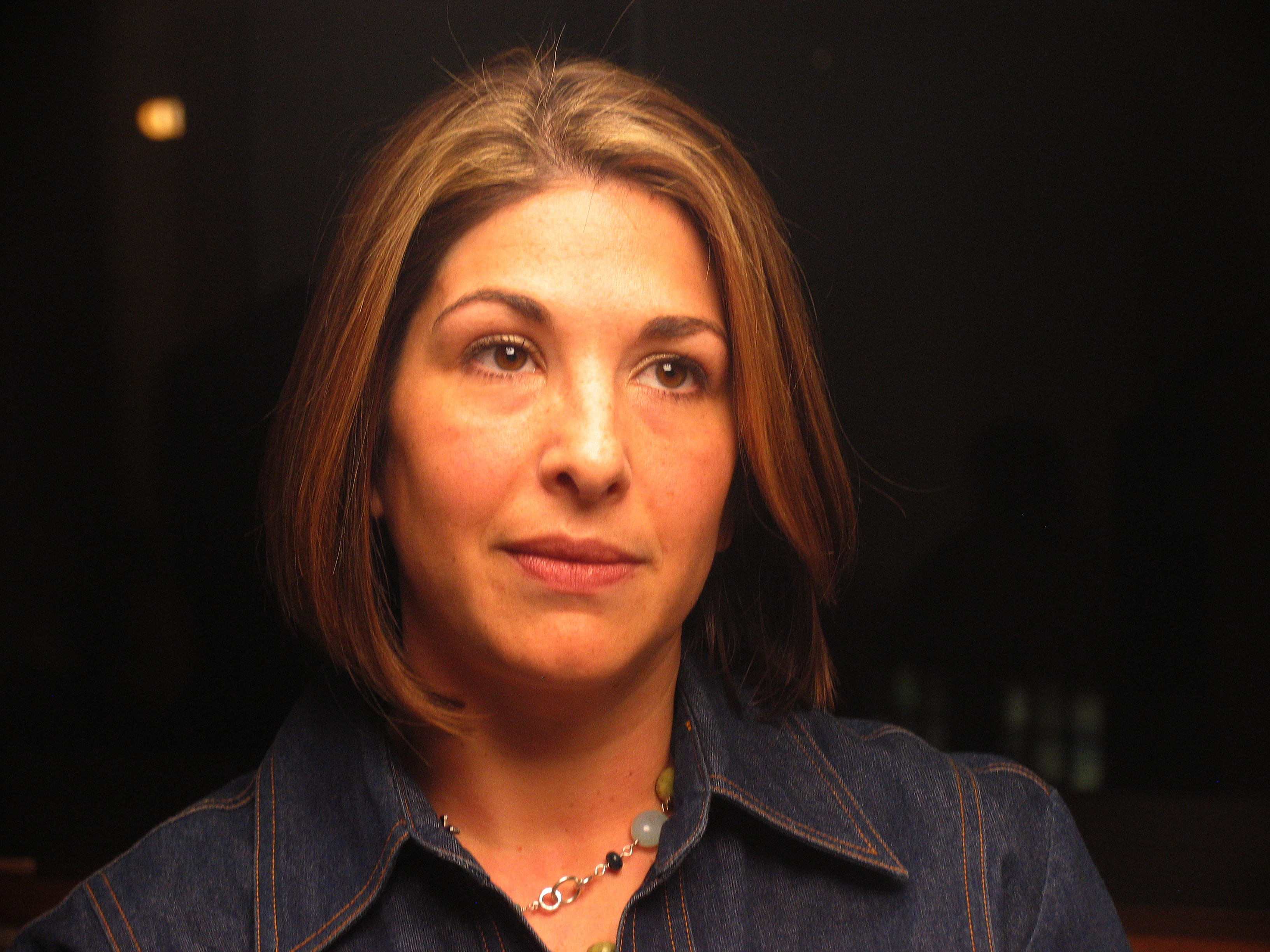This photograph features a close-up of a woman taken from the upper chest upwards, focused primarily on her face and shoulders. She has shoulder-length, straight brown hair with subtle highlights, parted slightly in the middle, and a few flyaways at the top. Her expressive brown eyes are accentuated with a touch of mascara, while her lips, adorned with light pink lipstick, form a slight, contemplative half-smile. She has thin eyebrows and her head is tilted slightly to the right, looking somewhat upwards and off into the distance. Her attire includes a blue jean jacket detailed with brown stitching, and around her neck, she wears a loosely draped silver necklace adorned with black, brownish, and blue-green translucent beads. The background is predominantly black, creating a stark contrast with the subject, though faint white squares and a pronounced yellow light in the top left corner add subtle depth to the scene.